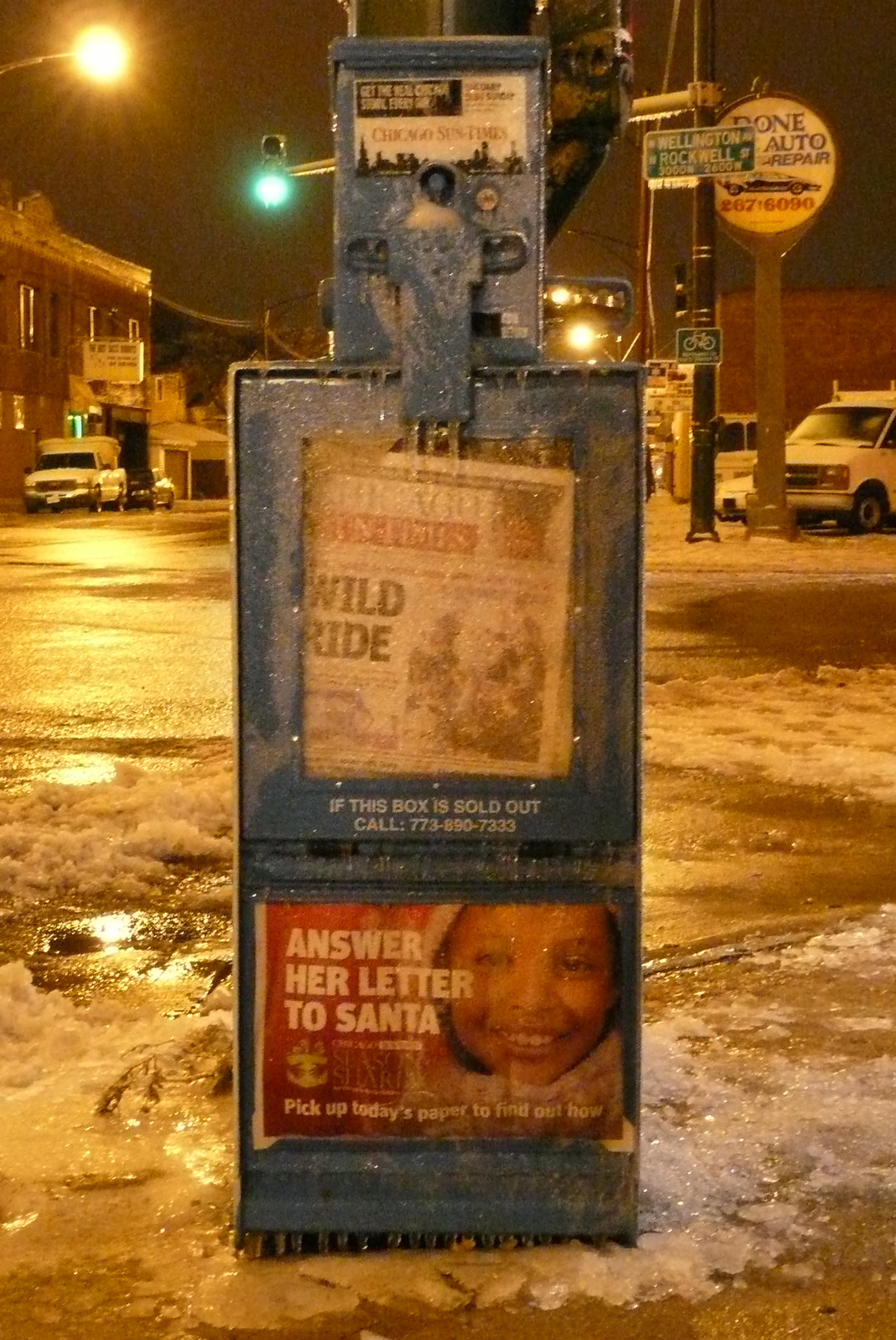In this image, we see an icy blue newspaper vending machine, prominently displaying the "Chicago Sun-Times" logo at the top. The machine, divided into an upper and lower section, is heavily covered in frost, icicles, and snow, indicative of the very cold and snowy conditions. Inside the upper half, a newspaper with the headline "Wild Ride" is visible against the frost-encrusted window. The lower half features an advertisement with a smiling girl and the words "Answer her letter to Santa." Surrounding the machine, the scene depicts an early morning street corner, with dark skies signaling the pre-dawn hours. To the right, there's a road sign reading "Wellington Ave" and "Rockwell St," alongside a circular white sign with blue lettering for "Done Auto Repair." The backdrop includes a brick building on the left, partially obscured by a white truck parked on the slushy, snow-covered roadway. Additional details like an ice machine and the general ambiance of a frigid, frozen environment frame this snapshot of a wintery urban street.